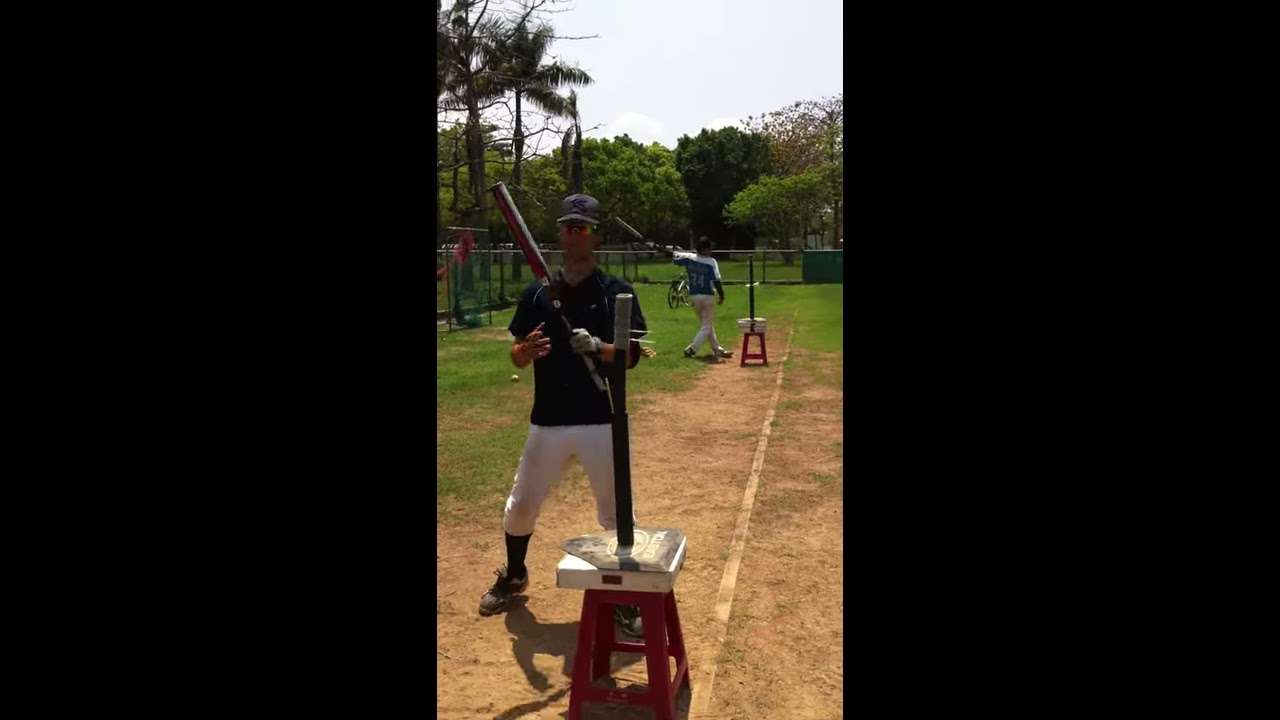The image features a scene of two young adults practicing baseball on a sunny day in a park. The composition is divided into three vertical rectangles; the first and the last rectangles are entirely black, framing the detailed central section. In the middle, the primary focus is a man facing the camera, grasping a baseball bat in his right hand. He is attired in a navy short-sleeved shirt, white pants, knee-high black socks, black shoes, and a dark blue baseball cap. In front of him, there is a red stool with a black vertical stick positioned on top, seemingly intended for batting practice.

In the background, another individual, similarly dressed in a blue and white uniform, has just completed a swing with his bat, his left arm extended backward. They stand on a grassy field, which appears slightly faded, bounded by a chain-link fence. Behind the players, a lush backdrop of trees and patches of grass can be seen, along with hints of houses and possibly a park feature. The scene is bathed in daylight, with clear blue skies overhead, indicating a warm and sunny summer day.